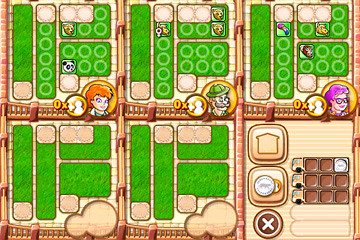This screenshot depicts a simplistic, low-quality animated video game likely designed for smartphones. The game features an adventure-type farming theme with several green, rectangular plots arranged in grids, each displaying various white circles and stretches of green, signifying crops or growth stages. The scene includes three distinct characters assigned to the top-row plots: a pale-skinned individual with red hair and a panda and bear icon beside them, a mustachioed man with a green hat portrayed alongside a penny icon, and a pale-skinned female character with purple hair and glasses, also accompanied by a penny icon. 

In total, there are six square blocks, each containing smaller rectangular green areas with white circles or entire white sections. At the bottom right, there's a utility area featuring a house icon, a coin, and an X button to close the menu. The image's pixelated details and the basic features of the characters indicate the game’s minimal graphical quality, contrasting sharply with richly detailed visuals seen in advanced gaming consoles.